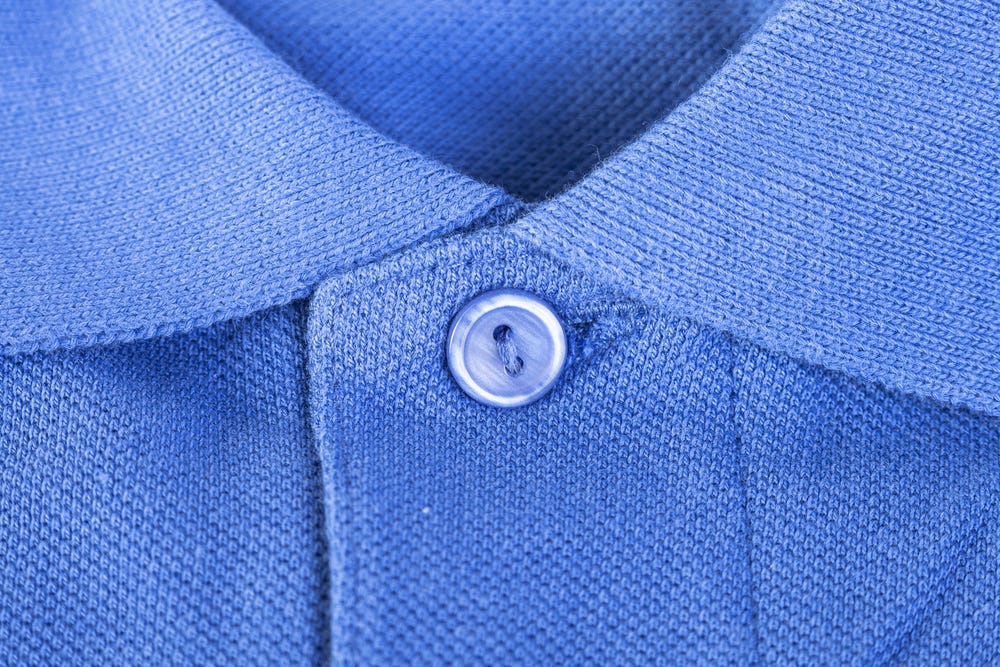The photograph is a horizontally aligned rectangular close-up of the collar of a blue polo shirt, focusing centrally on a single, shiny blue plastic button. The button, which has two holes, is secured with blue thread and is fastening the turned-down collar of the polo shirt. The fabric of the shirt is thick, likely a polyester blend, with a subtle zigzag textured pattern. The visible portion of the shirt includes both edges of the collar on the left and right, the top section of the shirt, and the strip where the button is attached. The light blue color of the garment is consistent throughout the visible area, which includes portions of the back and the collar. Though not visible in the image, the positioning suggests the potential location of the shirt tag just above the frame. The shirt appears to be laid out flat, allowing a clear and detailed view of the button and collar.